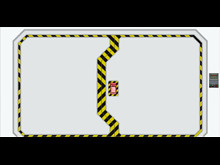A screenshot of a minimalistic, retro-style game is depicted. The game's interface is framed by black bars at the top and bottom of the screen, providing a stark contrast to the simplistic design of the game's visuals. At the center, a red car is positioned on a gray track. The track is outlined by a distinct yellow caution line, which not only encompasses the entire circuit but also traverses through it, creating a hazardous path. The left and right borders of the screen are open, blending into the track's background color. On the right side of the screen, there is a small element that resembles a slider, situated midway up the interface. The overall aesthetic and primitive graphics suggest that this is a capture from an old, very simplistic game, evocative of early gaming eras.